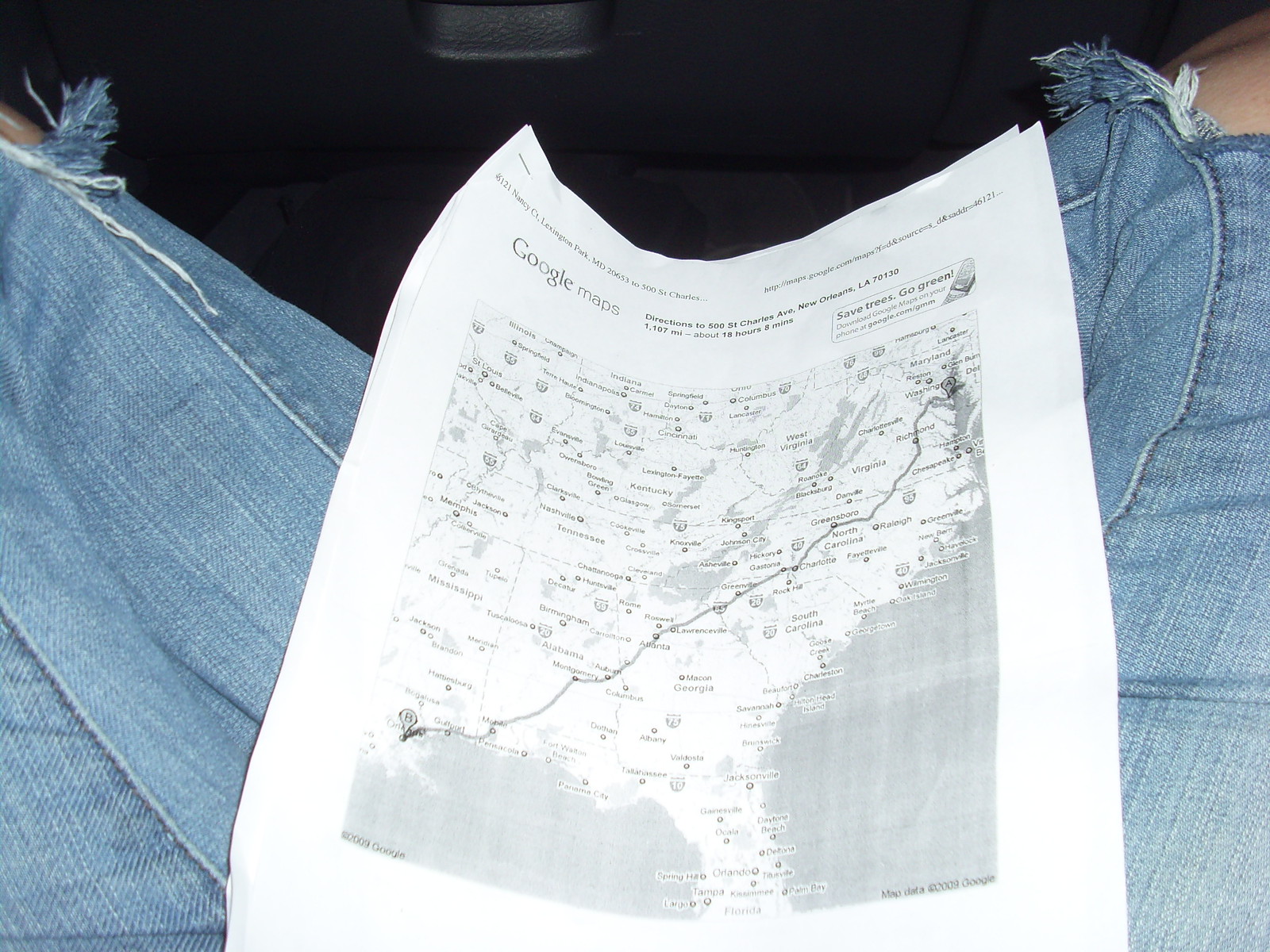The image features a color photo of an individual seated, likely in a vehicle, with a printout from Google Maps resting on their lap. The printout, which appears to be in black and white, displays a route that starts somewhere in Texas and heads towards the northeastern United States, with regions like Maryland, Georgia, and Florida visible. The map, including the Google Maps logo at the top, is centrally placed on the person’s lap, flanked by a white perimeter. The individual is wearing very faded blue jeans, with the knees torn and revealing caucasian skin. The person's legs are positioned in a V shape, extending towards the left and right, and the black background suggests they might be on a road trip. Despite the visible route details and the overall map layout, the exact starting and ending points, as well as the person's gender, remain ambiguous.